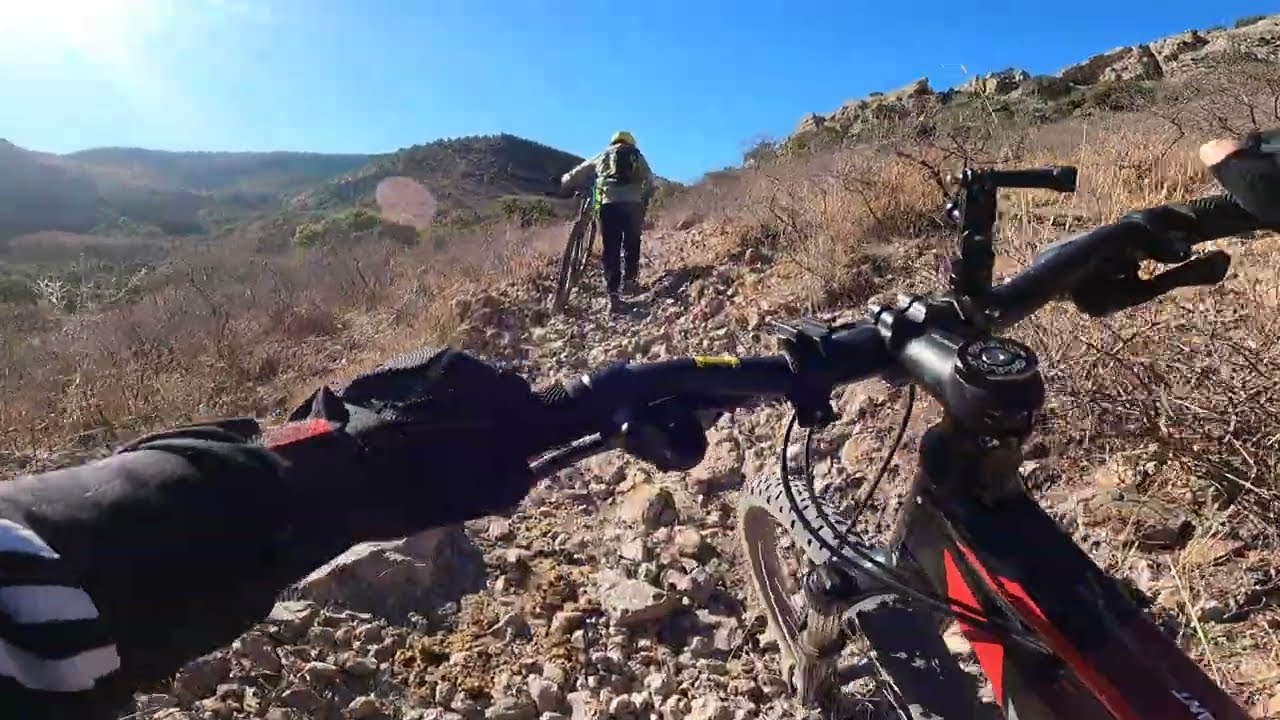The photograph captures the point of view of someone walking their black and red bicycle along a rugged dirt path filled with large and small rocks, sticks, and other outdoor debris. The person navigating this rocky terrain wears black gloves with a hint of red above the wrist, and their black and gray striped sleeve can be seen on the left handlebar, while the right handlebar is just outside the frame. In the background, another individual, clad in dark pants, a sage green jacket, a backpack, and possibly a white helmet, walks alongside their bicycle. This second cyclist is positioned towards the center left of the image, moving away from the camera. The landscape shows rolling hills and rugged terrain extending to the top right, with dried brush and sticks scattered across the scene. Above, the sky is a clear blue, and the bright rays of the sun beam down from the top left corner, highlighting the challenging and sunlit path ahead.